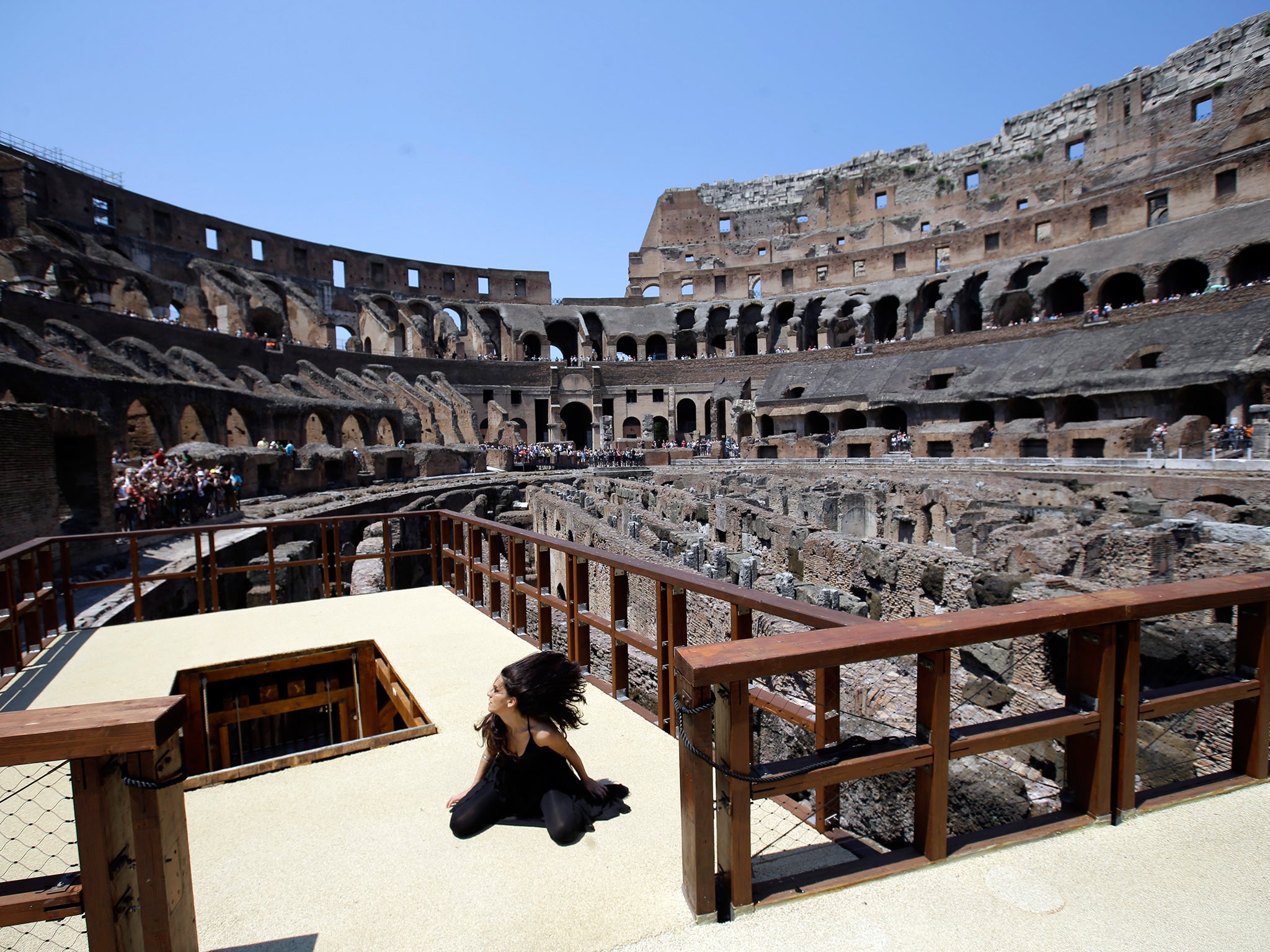The image captures a professional photograph taken inside an ancient, weathered arena, likely the Colosseum in Rome. In the foreground, a female model with flowing black hair is striking a delicate pose on a white cement platform set up for tourists. She is dressed in a sleek black pantsuit, kneeling with her hands resting on her feet, gazing contemplatively to her right. The background reveals the multi-tiered interior of the Colosseum, composed of mottled, deteriorating stone in shades of brownish-gray, with visible holes and crumbling sections. Around the platform are wooden railings and brown fence posts, while hints of tourists in colorful outfits can be seen meandering along the various levels. The sky above is a clear blue, adding to the daytime setting of this striking and evocative scene.